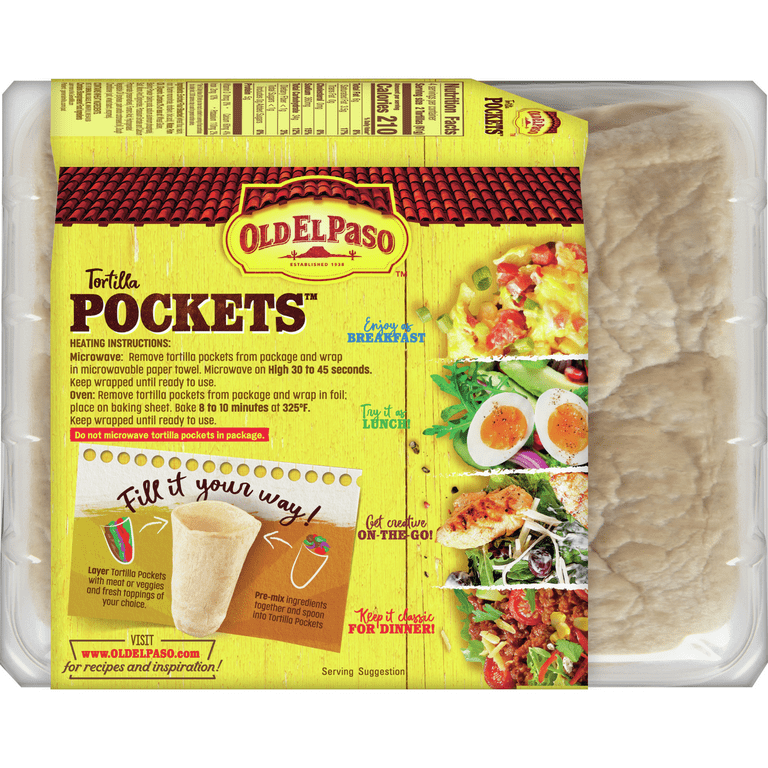This image features a photograph of an Old El Paso brand tortilla pockets package, displayed in a horizontal rectangle format with slight protrusions at the corners. The package is encased in clear plastic wrap, through which the tortillas are visible on the right side. Overlaid on the plastic is the box cover, slightly bent at the top, revealing the Old El Paso logo set against a bright yellow background, styled to mimic a Spanish ceramic roof. The left side of the box highlights the product name; "tortilla" is in cursive, while "pockets" is prominently displayed in large brown letters. Beneath this, various lines of text offer heating instructions and serving suggestions.

The box cover creatively illustrates different meal ideas organized by time of day, each accompanied by small white and color-coded text. At the top, "Enjoy your breakfast" is paired with an image of an egg mix. Below that, "Try it for lunch" features a salad, followed by "Get creative on the go" showcasing what appears to be a chicken salad. The bottom suggestion, "Keep it classic for dinner," displays a traditional taco filling. Additional text directs consumers to visit OldElPaso.com for recipes and inspiration. The box sleeve, with nutritional information visible on the side, lays atop the plastic-wrapped tortillas, extending slightly over the edges on the right side.